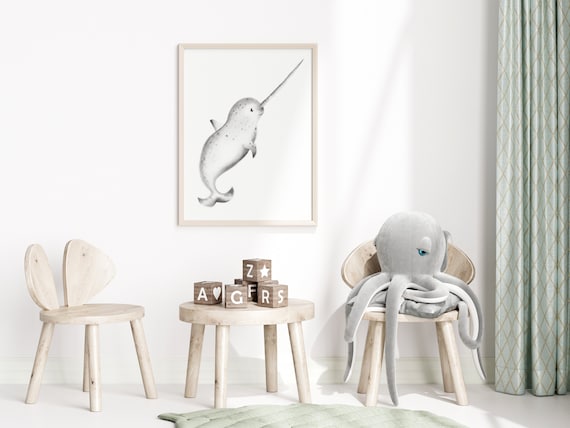This is a detailed image of a child's modern and bright bedroom featuring light wood furniture and mint green accents. Central to the room is a small table flanked by two matching light wood chairs with plain peg legs, all arranged on a green rug. One of the chairs hosts a large stuffed octopus toy, its tentacles draping down. The table is adorned with wooden letter blocks displaying letters such as A, G, Z, F, R, and S, alongside shapes like stars and hearts. Behind the table stands a white-framed painting of a narwhal on the white wall, which is bordered by a green curtain with a diamond zigzag pattern. Despite the playful elements, the room maintains a serene and minimalist aesthetic with its soft, neutral tones.